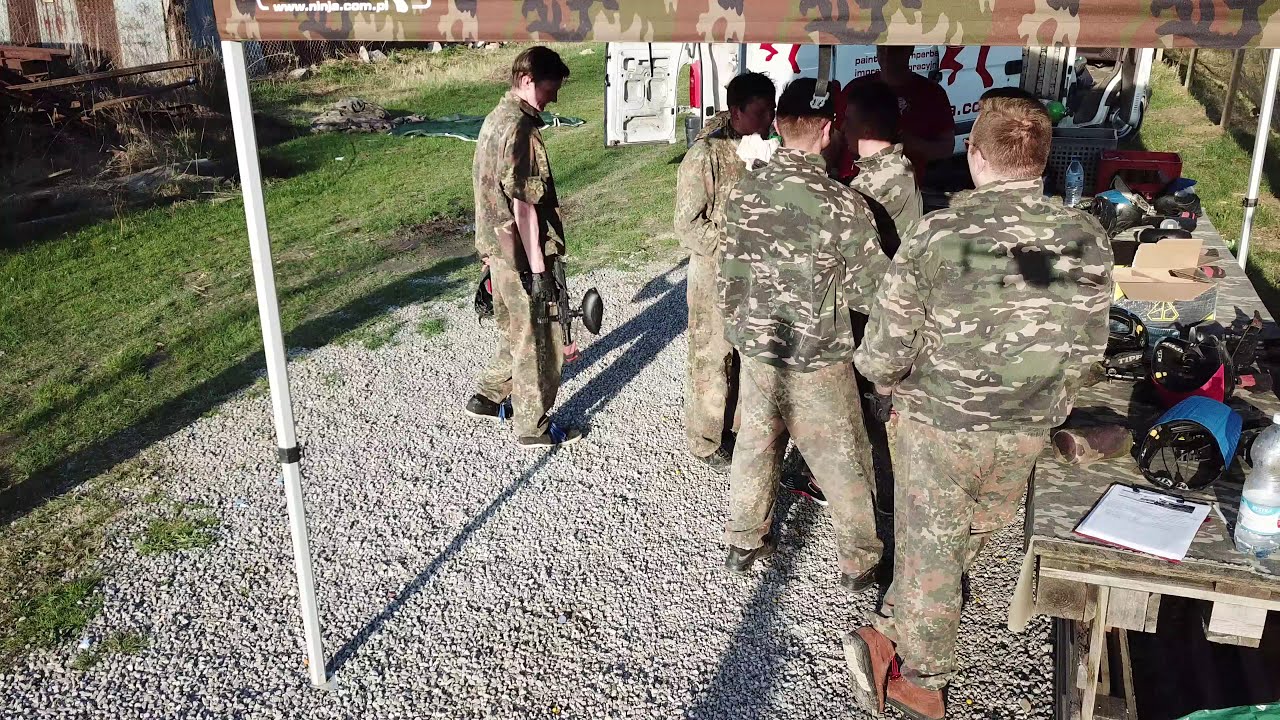The photograph captures an outdoor military training activity or a paintball session under natural daylight. In the foreground to the right, there is a section of crushed gravel and white stone ground. A group of six individuals, all dressed in camouflage outfits consisting of jackets and trousers, stand with their backs to the camera. A shadowy figure appears to be addressing them.

In the background, a white van with red designs and some text on one of its rear doors stands with a door open. To the left of the group, there is a table covered with camouflage fabric, displaying various paintball gear including masks, bottles of water, boxes, and even a clipboard.

One of the individuals is holding a black paintball gun and a mask, while another, dressed in camouflage gear with rolled-up sleeves and black trainers, stands looking down. Additionally, another camouflaged individual with brown shoes and glasses leans against the table. The scene is framed by a camouflage canopy overhead, featuring text in the top corner that reads "www.ninja.com.pl." To the left of the gravel area is neatly cut grass, with some buildings and structures visible in the image's top left corner.